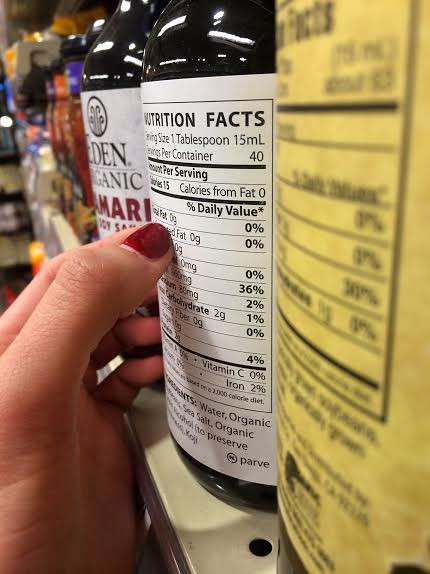This close-up photograph captures a row of various bottles, likely wine, arranged on white utilitarian metal shelving, extending into the distance on the upper left side. The composition focuses intently on one bottle with a white nutritional information label, which is being touched by a person's left hand. The hand, characterized by white skin and fingernails painted a striking burgundy or red color, has the thumb resting on the label and the bottoms of their fingers visible from the palm side. The label features black lettering and details such as "nutritional facts." The bottle in question is black, flanked by a green-labeled bottle on one side and a white-labeled bottle on the other. The prominent nutritional facts include "calories from fat is zero," and "calories per serving is 15." The hand's positioning suggests the person is reading and pointing at specific lines of the nutrition facts, indicative of a discerning review of the contents. The scene appears to be situated in a grocery store, amidst a backdrop of varied colors including purples, reds, yellows, and oranges.